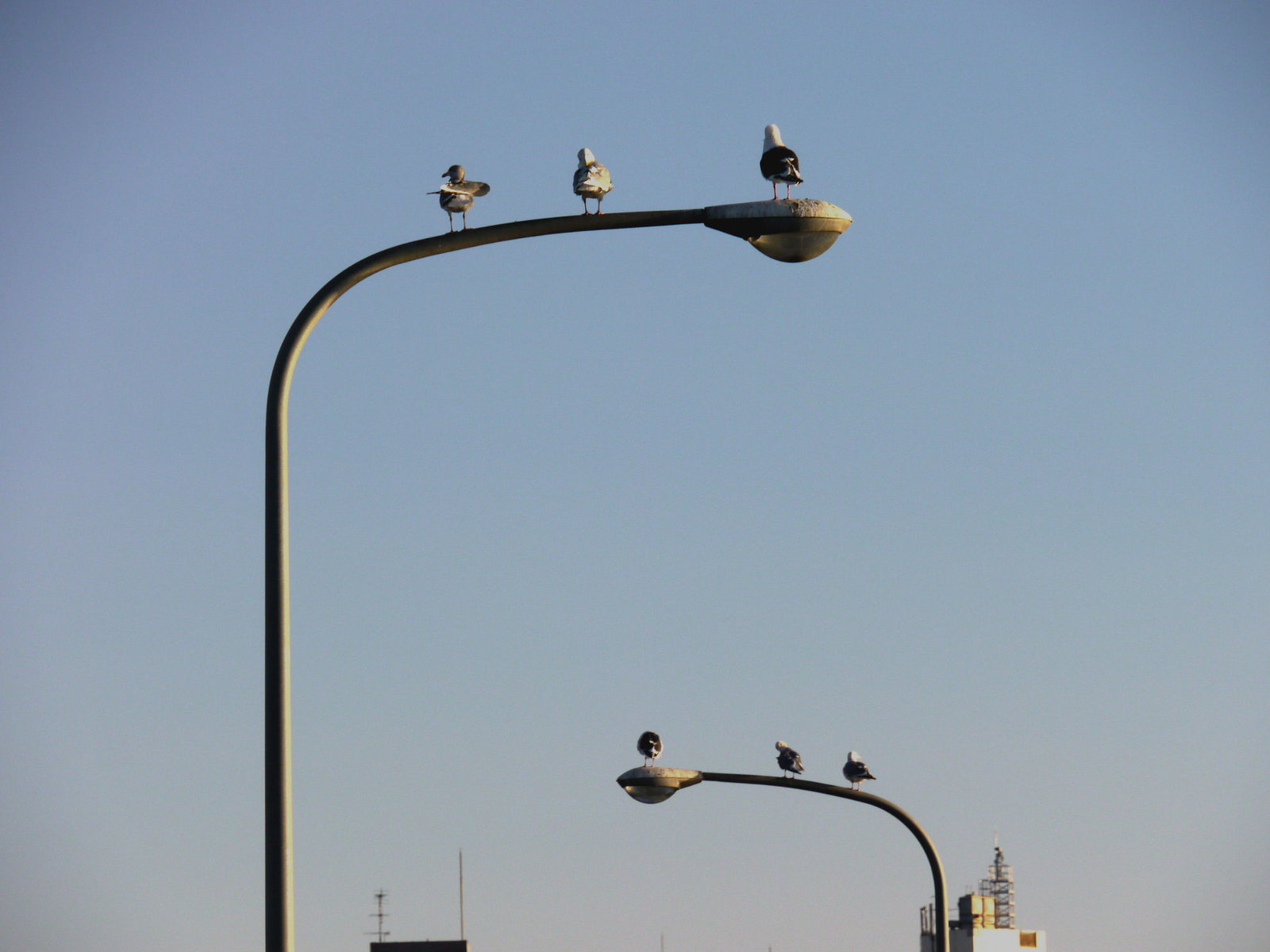In this outdoor photograph, a clear blue sky gradient serves as a serene backdrop, from a darker blue at the top to a lighter blue near the horizon. Two city street lights, each with a classic dome-shaped light fixture that remains off during the daytime, feature prominently in the composition. One street light is positioned near the top of the image, and the other near the bottom right.

Perched on each street light are three birds with slender legs. On the top street light, two birds have white fluffy heads and black bodies, while the third bird sports a darker head and coat with a white tail. One of these birds appears to have its wings spread out. On the lower street light, the perched birds include one entirely black bird, a black and white bird, and another with a white head and a darker coat. 

The birds all gaze off into the distance, adding to the tranquil scene. At the bottom of the photo, the tops of tall, industrial-looking buildings are visible, adorned with a few poles protruding from their rooftops. The gray poles of the street lights and the slight haze in the sky contribute to the city's urban aesthetic.